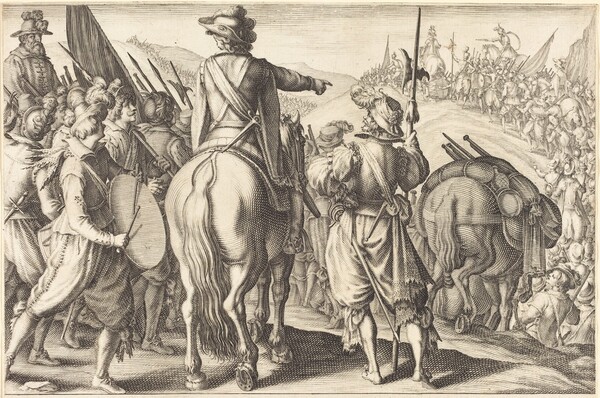This black and white ink drawing, rendered with intricate detail, depicts a historical army preparing for battle. The composition features numerous soldiers, many on horseback, wearing military uniforms and carrying shields and packs. Central to the image is a commanding figure on horseback, pointing decisively to the right, indicating the direction of their impending journey. Adjacent to him, another figure is depicted mid-stride, beating a drum. In the forefront, the tops of weapons can be seen, adding to the anticipation of an imminent battle. The entire scene is characterized by a monochromatic palette, primarily black ink on an off-white background, with hints of tan evoking a sense of age. The depiction includes various horses burdened with supplies, emphasizing the logistical preparation for the voyage. The perspective appears to be from behind the army, allowing a view of the procession moving along a path that ascends slightly, suggesting a rugged terrain. The drawing's style and the historical military theme contribute to the impression of a bygone era.